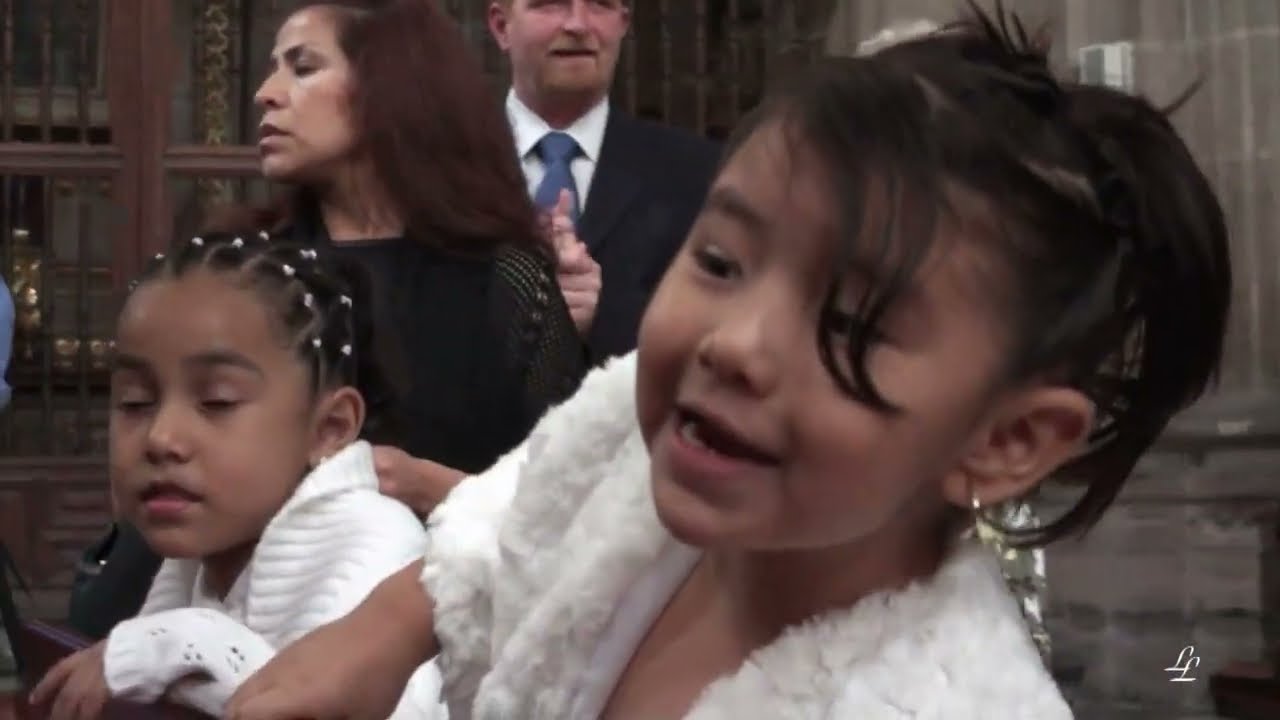The image depicts a scene with two young girls in the foreground and a man and woman in the background, all dressed elegantly. The girl on the left in the bottom part of the image has black braided hair adorned with white decorations and is wearing a white sweater. She has a slight smile and her eyes are partially closed, looking forward and slightly to the left. The girl on the right has unbraided black hair that falls into her left eye and is also wearing a white short-sleeved dress. She, too, is looking to the left and is smiling. Behind the girls, to the upper left, stands a man in a black suit with a blue tie, and next to him, a woman in a black dress with long reddish-brown hair. The man appears to be looking straight ahead while the woman gazes to the left. The background features a wooden wall with multiple windows and white curtains, though parts of it are blurred. In the bottom right corner of the image, there is a logo "LL". The overall setting is bright and clear, emphasizing the formal attire and setting of the individuals.